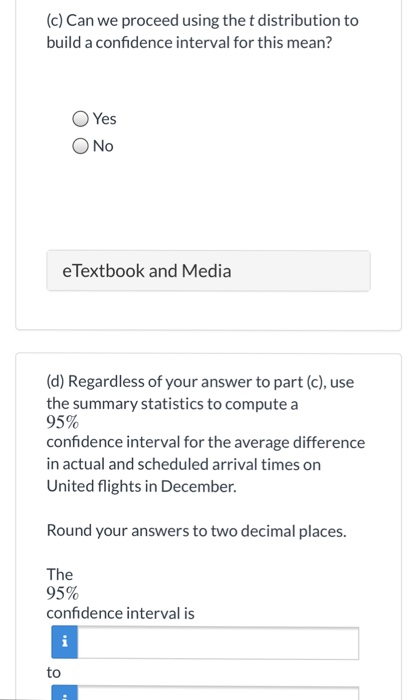Image Description: The image comprises screen captures of two question frames, each framed in either a square or a rectangular shape with a white background. The top question frame is inscribed with black text, reading:

"Let us see. Can we proceed using the t-distribution to build a confidence interval for this mean?" 

Below this question, there are two selectable options displayed: "Yes" or "No." Beneath these options, a pale gray frame contains black text that reads: "e-textbook and media."

The second question frame, situated below the first, also features black text. It states:

"D. Regardless of your answer to part C, use the summary statistics to compute a 95% confidence interval for the average difference in actual and scheduled arrival times on United flights in December."